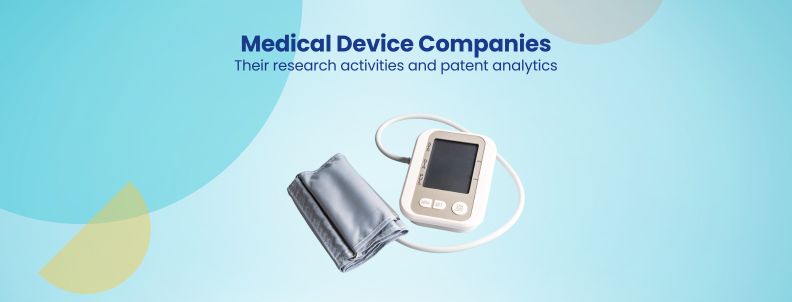The image appears to be a promotional webpage for medical device companies, highlighting their research activities and patent analytics. Centered prominently in the image is a medical device—an automatic blood pressure monitor, consisting of a white base unit with a screen and an attached grayish-blue cuff, designed for home use. The background features a soothing blue color scheme, accentuated with darker blue bubbles and two semicircles, one yellow and one gray, adding a visually appealing touch.